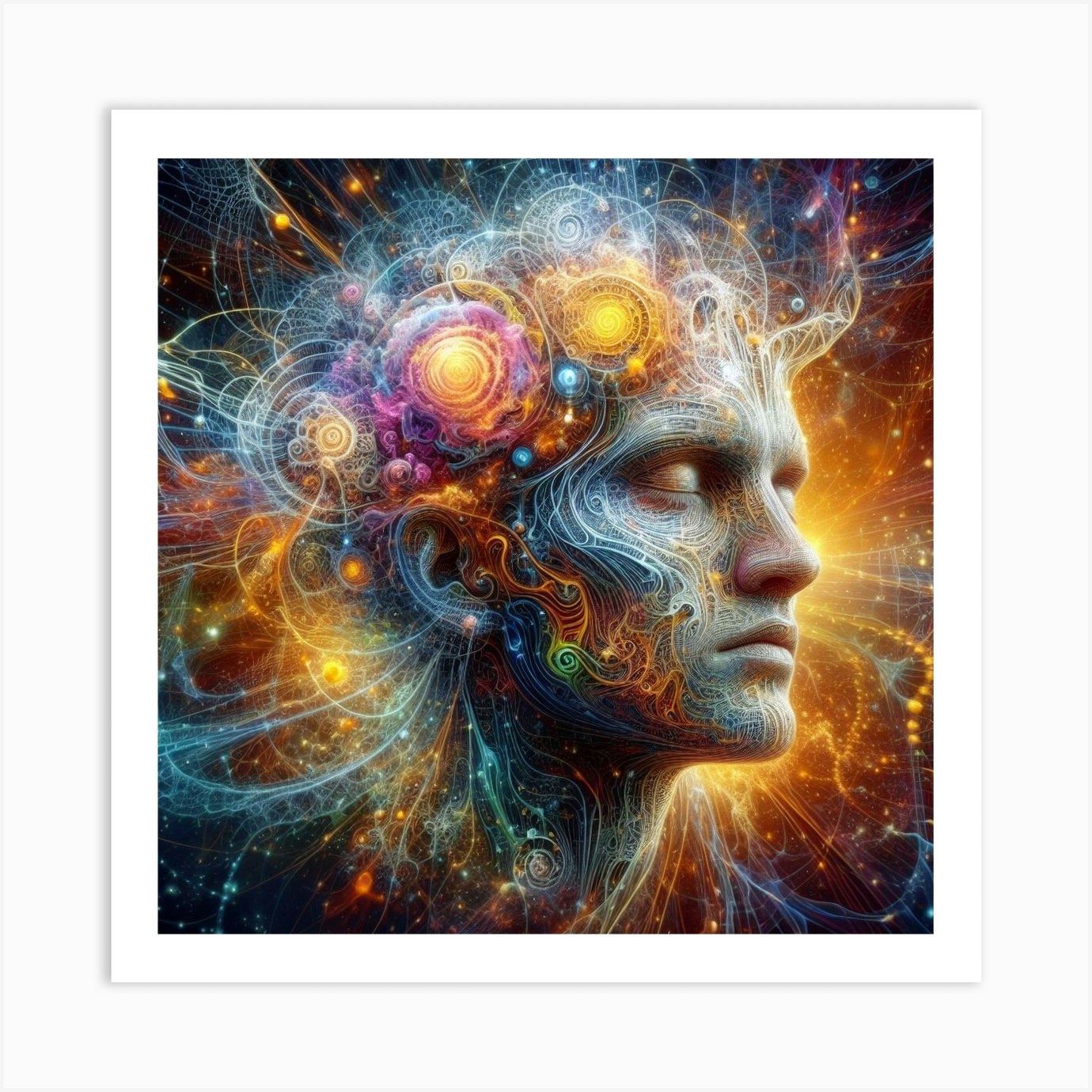The image showcases a large, AI-generated portrait hung prominently on a white wall. The face, depicted in an almost blueprint-like, technological manner, features closed eyes, a visible ear, and a neck, all oriented in a side profile. The central face is engulfed in a mesmerizing array of colorful, swirling lines that evoke a sense of cosmic energy. Particularly striking are the two golden, circular patterns that spiral into each other on the sides of the head, surrounded by a mix of white, purple, and golden hues. The hair is rendered as an intricate web of white swirls radiating in all directions. The upper corners of the image are tinged with a darker background, speckled with tiny blue stars, giving a celestial impression, almost as if the portrait is set in a starry sky. The entire composition emanates an orange glow from the background, contributing to its vibrant and ethereal quality.